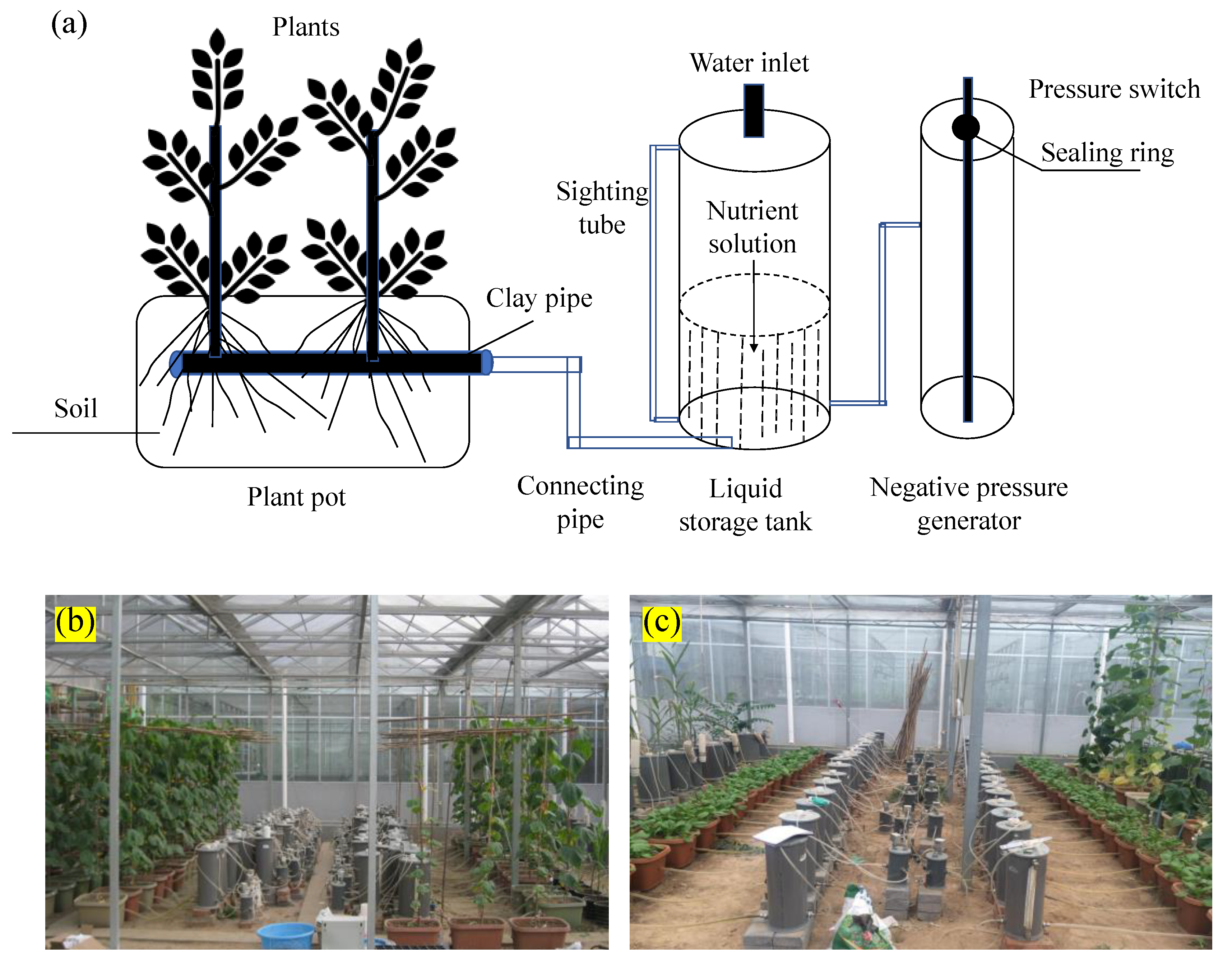A detailed diagram and photograph set illustrating a complex plant growth setup. At the top, a blueprint-like drawing, primarily in black and blue, meticulously labels various components essential for plant cultivation, such as “plant,” “soil,” “plant pot,” and “clay pipe,” along with mechanisms like “water inlet,” “siding tube,” “connecting pipe,” “nutrient solution,” “liquid storage tank,” “pressure switch,” “sealing ring,” and “negative pressure generator.” The detailed diagram connects these parts visually, showing their integration into the system.

Below, two color photographs labeled B and C depict the real-life application of the diagram within a greenhouse setting. Photograph B showcases green plants in clay, white, and blue pots, silver canisters connected by tubes, and additional plants to the right side, all set on a dirt floor. Photograph C displays shorter plants within pots and canisters connected through tubing, arranged similarly with a central array of silver cylinders and more plants on either side. The photographs provide a vivid, side-by-side comparison of the diagram’s concepts in practical, real-world scenarios, capturing the structured environment of a working greenhouse. The use of black and blue in the drawing contrasts with the vibrant photos below, enhancing the understanding of the setup and its components.